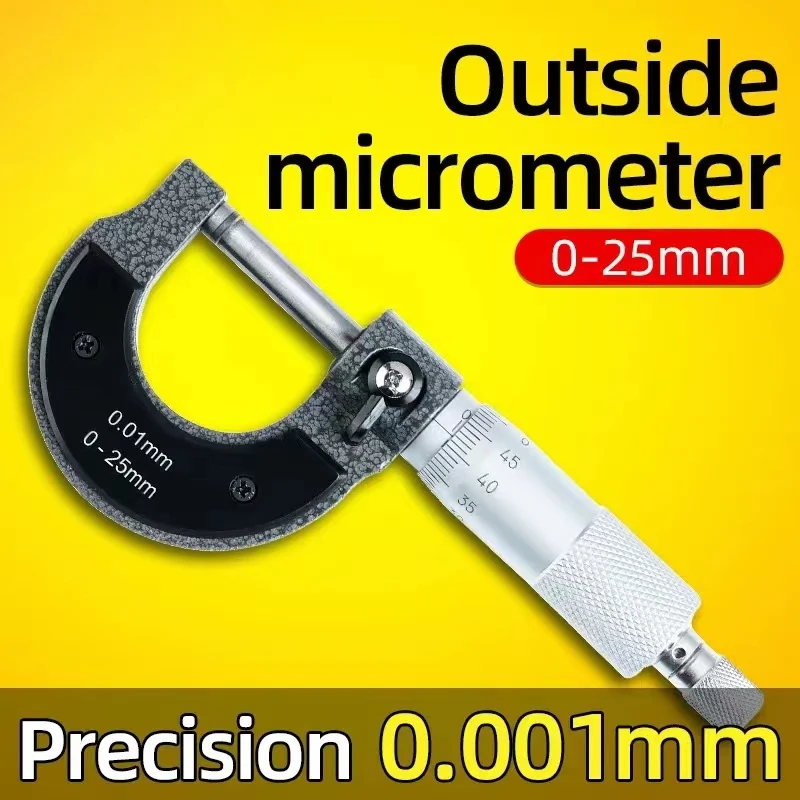The image is a detailed product advertisement for an outside micrometer, prominently set against a yellow background. The micrometer itself has a metallic handle with a cylindrical dial on the side featuring dashes and numbers for precise measurement adjustments. This dial ranges from 0.01 mm to 0.25 mm, enhancing its precision. Attached to the handle is a rounded, black and gray horseshoe-shaped clamp with an interior metal rod that facilitates the clamping mechanism. 

At the top of the image, black font text reads "Outside Micrometer," followed by a small red oval with white font indicating the measurement range "0 to 25 mm." A brown-tinted banner at the bottom includes white text that says "precision," with yellow font specifying "0.001 mm," underscoring the device's high degree of accuracy. This detailed image emphasizes key features of the outside micrometer, making it easily identifiable for those seeking precise measurement tools.